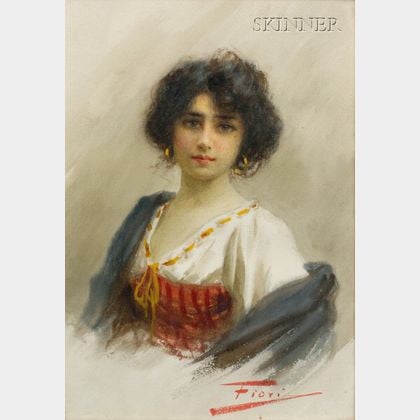This detailed portrait captures a beautiful woman with a serene expression. Her face, depicted with pale white skin and rosy red cheeks, is framed by her curly black hair that just touches her ears. She is adorned with gold hoop earrings and has bright pink lips that add a touch of vibrant color to her fair complexion. Her outfit features a white blouse with an intricate red lace detail around the chest, complemented by a red corset. She also wears a light gray knit sweater draped casually over her shoulders. Adding to her appearance, the blouse has gold stitching on the collar, enhancing its elegance. 

The portrait is signed by the artist 'Fiori' in red text at the bottom right corner, while the top right corner bears the caption 'Skinner.' The background of the painting is primarily white with subtle gray shading, setting a neutral stage for the woman's striking features. The woman gazes straightforwardly at the viewer, her look calm and composed, as though resting. This delicate and well-crafted artwork, with its understated yet meticulous details, leaves a lasting impression of grace and beauty.